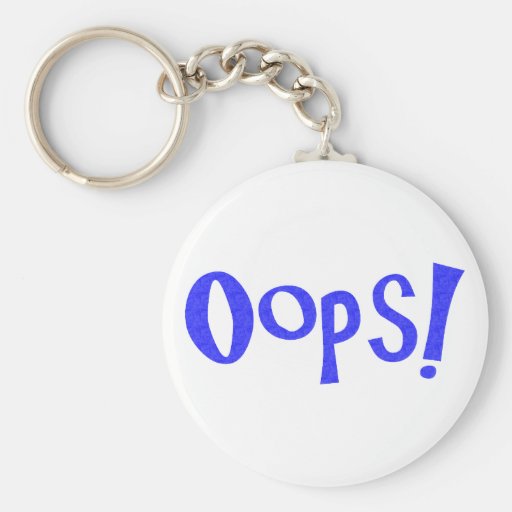The image showcases a square photograph featuring a silver keychain set against a very light cream or off-white background. The keychain's notable elements include a round metallic loop positioned in the upper left corner, which connects to a short chain composed of five oval links. This chain leads diagonally to the bottom right corner of the image, where it attaches to a circular white pendant. Prominently displayed in blue lettering on the pendant is the word "OOPS!" followed by an exclamation mark, centered within the white round shape. The simplicity of the scene and the keychain's placement create a clear, minimalist composition.